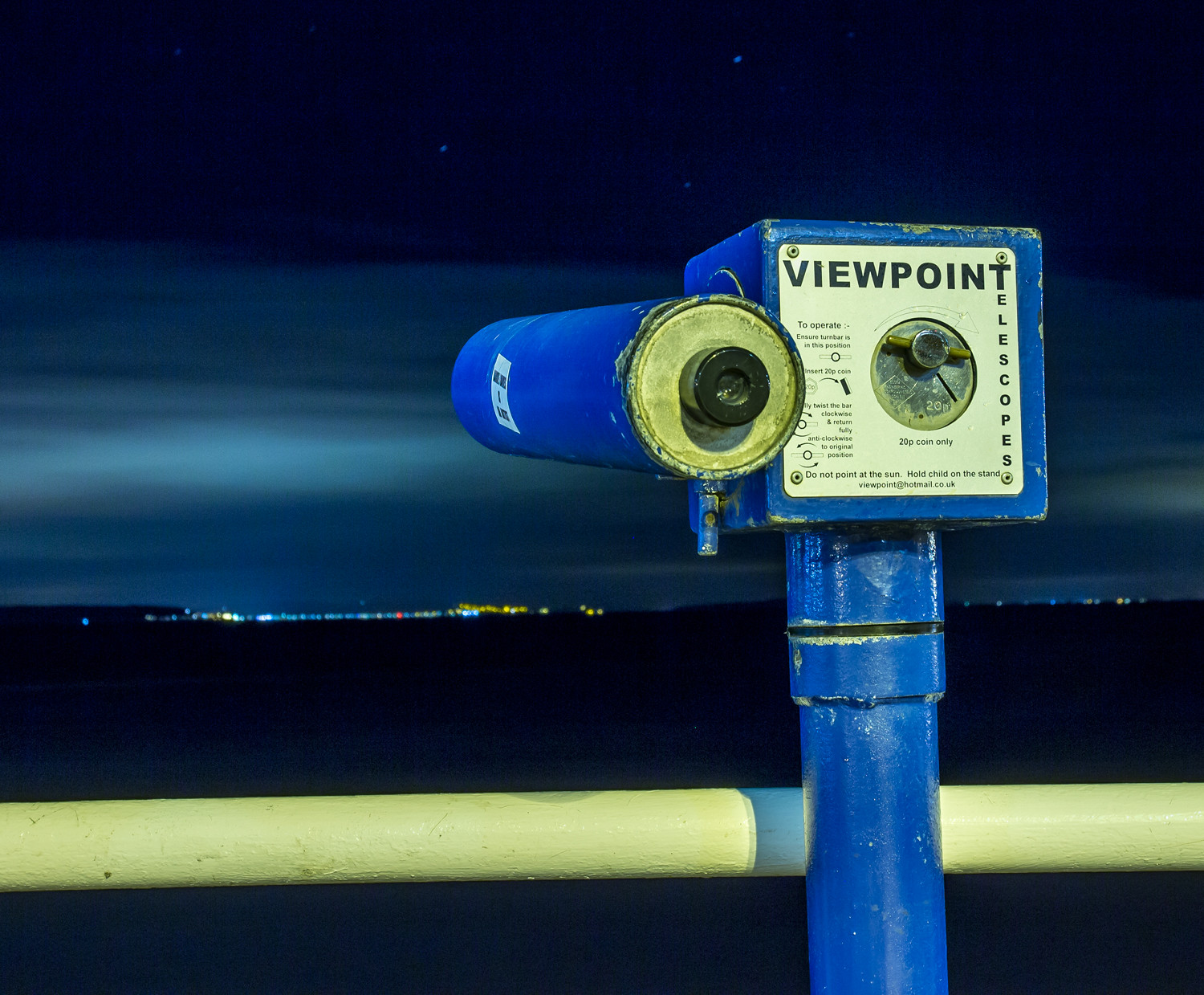The image depicts an outdoor viewing platform featuring a viewpoint telescope. Dominating the right-hand side of the image, this telescope is mounted atop a pole that rises from the platform, extending beyond the bottom frame of the picture. The telescope is affixed to a blue box, which prominently displays the word "Viewpoint" at the top in large black letters and smaller letters down the right side spelling "telescopes." The blue box also has an unreadable black text and a circular slot likely designed for coins. 

Flanking the blue box on the left is the telescope itself, which has a brass-encircled eyepiece protruding from its light-colored end. The device is set against a backdrop, which includes a white horizontal railing in the foreground. Beyond this railing, the scene transitions to a dark, indistinguishable area below, eventually revealing a distant cityscape awash with blurry, muted lights under a cloudy sky illuminated faintly, possibly by moonlight. The stars are faintly visible, adding a subtle celestial touch to the scene.